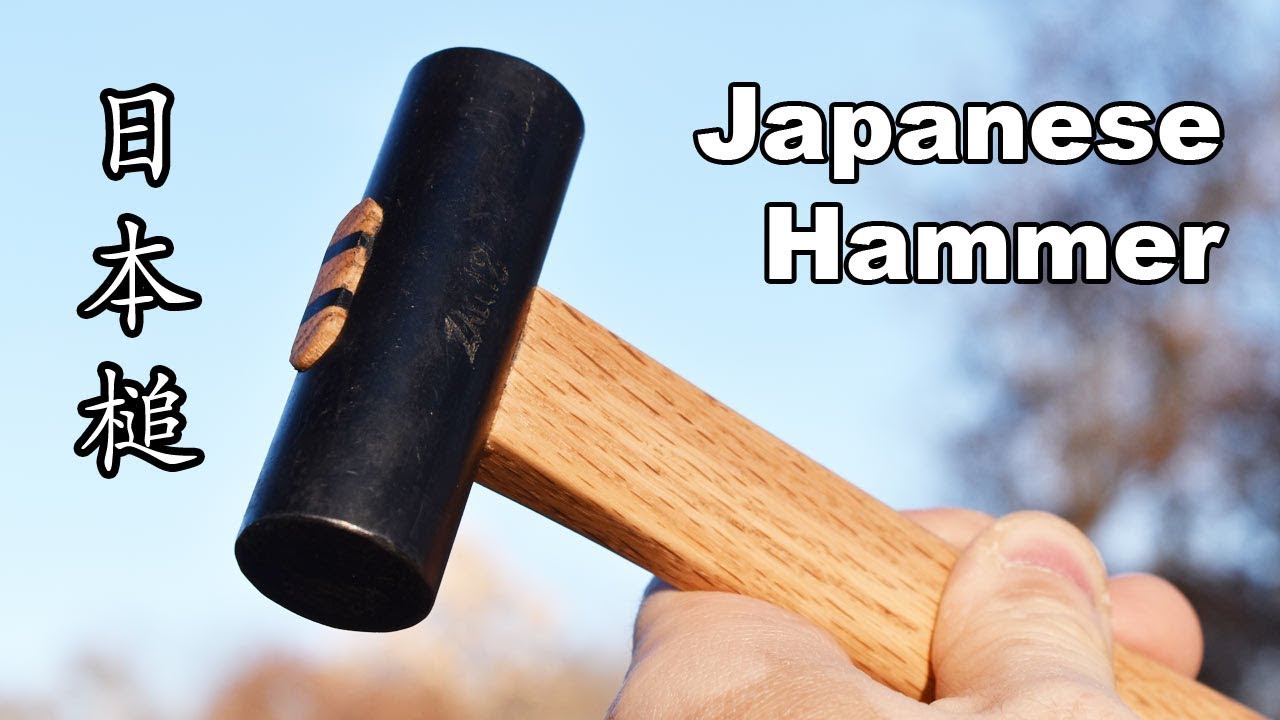The photograph, potentially a thumbnail for a YouTube video, features a centrally positioned black mallet-style hammer with a wooden handle, held by a man's left hand. The hammer head, which displays an inscription of indeterminate symbols in the middle, is predominantly black. To the left of the hammer, three vertically oriented white Japanese characters with black outlines are visible. On the right side of the image, large white text with a black outline spells "Japanese Hammer." The background is an outdoor setting with a pale blue sky and a large, blurred tree to the right, contributing to a serene atmosphere while emphasizing the focus on the hammer itself.